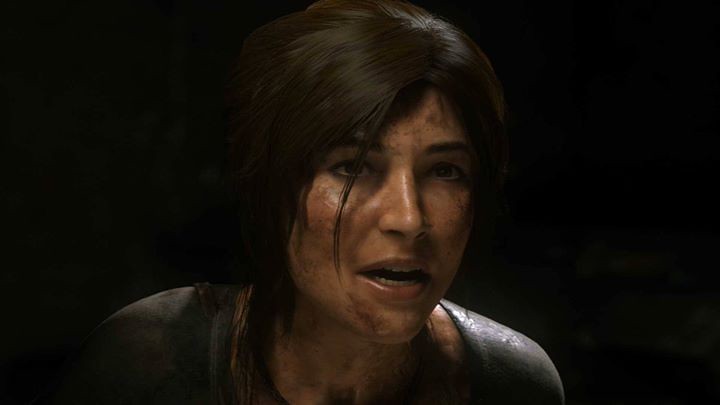This screenshot from a video game vividly captures a mid-aged woman with long, black hair and medium skin tone, dressed in a dirty outfit that appears greenish or dark blue. Her face is marked with dirt and possibly blood, highlighting the hardships she has endured. Her expression is one of shock and fear, with her mouth agape and her eyes staring off to the right of the viewer, suggesting a recent traumatic event. The background is predominantly black, with indistinct foliage visible on the back left side. The setting suggests a post-apocalyptic or horror-themed game, reminiscent of titles like "The Last of Us." There's a distinct sense of tension and survival conveyed through the detailed and well-lit rendering of the character.